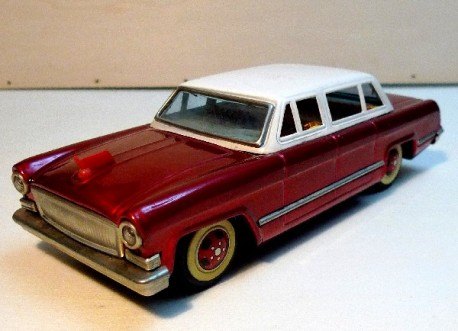The image features a small model car that appears to be from the 1940s or 1950s, set on a white surface with a beige wall behind it. The car is maroon wine in color, with wide white wall tires that have red rims. It has a distinctive long hood and a shorter rear, giving it a classic elongated shape. The front of the car features a solid, flat silver bumper, and the headlights are positioned under protruding bumps on the fenders. A chrome strip runs along the lower part of the car's sides. The roof and window frames are white, with the windshield being a straight sheet of glass, not curved. The car has front and back vent windows, adding to the vintage charm. The model is facing diagonally with its headlights pointing towards the lower left corner, casting a shadow. The image also reveals some wall details, such as nails, adding a touch of realism to the setting.